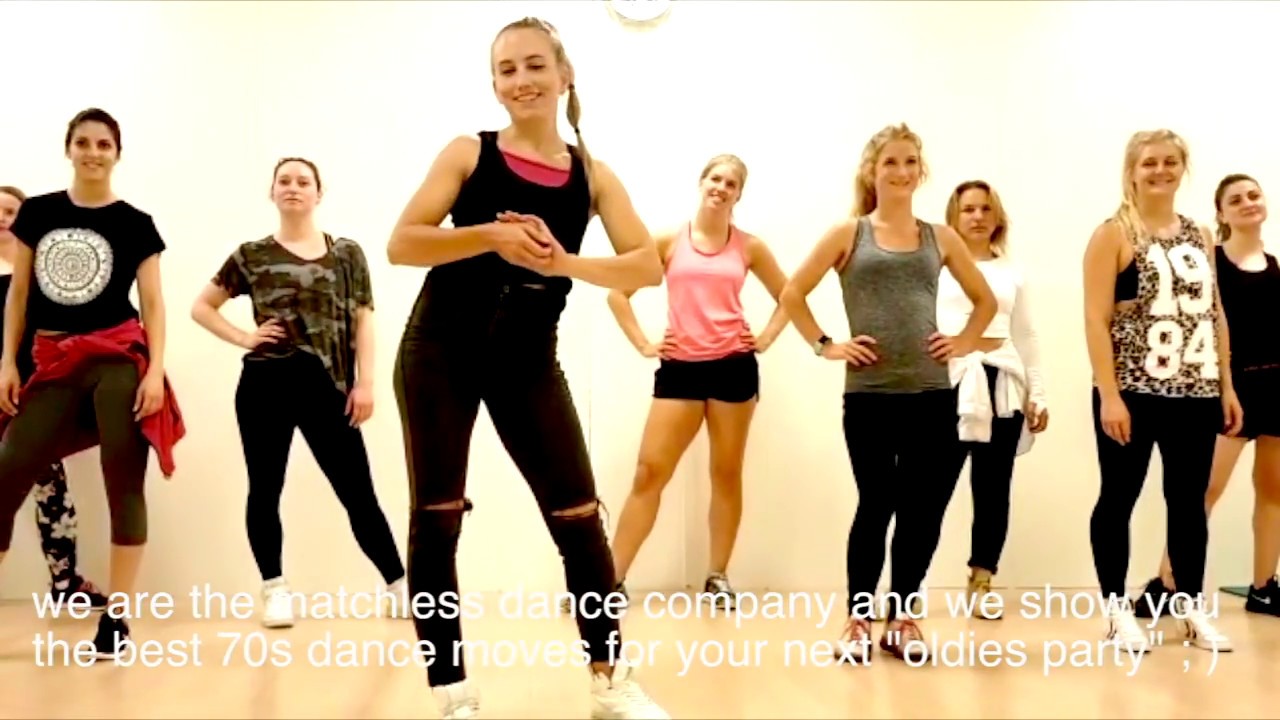The image depicts a lively scene of a group of women on a polished wooden floor, likely a dance studio or gymnasium, given the bright, white back wall with a subtle yellowish shadow. The wall features a prominent white lowercase inscription reading, "We are the Matchless Dance Company, and we show you the best 70s dance moves for your next 'Oldies' party."

In the foreground stands a woman who appears to be the instructor, her radiant smile enhancing the energetic atmosphere. She wears a pink tank top beneath a tight black sleeveless top, complementing her black pants and white tennis shoes. Her blonde hair is neatly pulled back into a ponytail that cascades over her shoulder. With her eyes closed and hips slightly angled to the left, she exudes confidence and joy.

To her immediate right is another woman, also smiling, who dons a pink tank top and short black shorts, revealing her long, white legs. Just right of center is another participant wearing a tight gray tank top and black pants, her hands poised on her hips.

Further to the right, a woman in a leopard-print tank top marked with the number "1984" stands out. She wears a black bra underneath, black tight pants, and white shoes, adding a touch of boldness to the scene.

There are a total of ten women visible in the frame, all dressed in various workout clothes and seemingly synchronized, possibly captured mid-dance or in preparation. The overall composition vividly conveys a dynamic dance class, poised to showcase vibrant 70s dance moves for an upcoming nostalgic party.